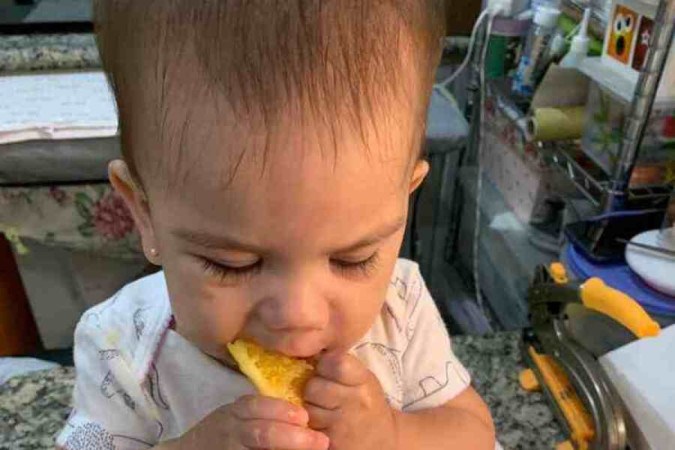The image captures a young, fair-skinned baby with golden wheat-colored hair and a small white pearl earring in the right ear. The baby, wearing a mostly white outfit with light purple and yellow designs, is seen holding an orange slice with both hands, eagerly sucking the juice out of it. The baby’s head is tilted downward, focusing on the task, thereby obscuring the eyes. The background is a visually cluttered scene featuring a packed storage shelf filled with various items like arts and crafts supplies, a roll of wrapping paper, a glue bottle, and a hand tool that resembles a hole puncher. Additionally, there are colorful objects and fabrics, including a piece of cloth with a red flower and green leaves, and something orange and black made of plastic and metal. The setting suggests this is likely within someone's home, amidst an environment rich with miscellaneous knickknacks and tools.